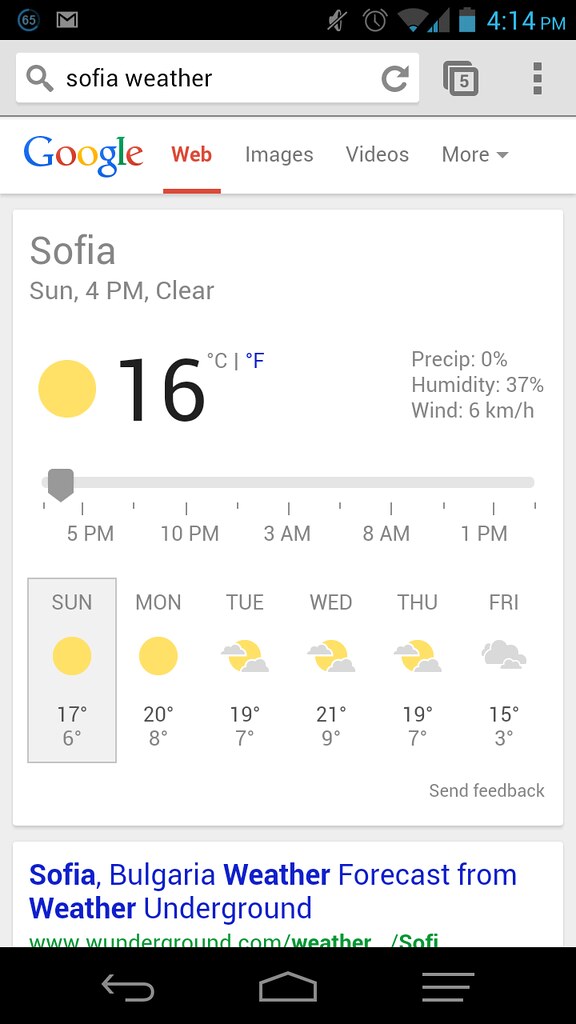The image is a screenshot from a tablet displaying a Google search result for "Sofia weather." The interface shows a typical weather forecast format provided by Weather Underground (www.wunderground.com/weather/Sofia). The screen is vertically oriented and has a white background. 

At the top of the interface, the multi-colored Google logo is prominently displayed in the upper left corner. The search query at the top of the screen reads "Sofia, S-O-F-I-A, weather," indicating the user is looking for weather information for Sofia, Bulgaria.

The main section of the screenshot features a detailed weather forecast. The top part of this section includes the heading "Sofia" along with the current date and time, presented as "Sunday, 4 p.m." The weather at that time is indicated as "clear," accompanied by a small icon of a sun representing the clear conditions.

Below this, the forecast extends for the next five days, from Sunday through Friday. The forecast summary is as follows:
- Sunday and Monday: Clear skies.
- Tuesday, Wednesday, and Thursday: Partly cloudy conditions.
- Friday: Completely cloudy.

The information is presented in a vertical layout, neatly organized within a rectangular box. This layout provides a clear and concise view of the weather predictions for Sofia over the specified period.